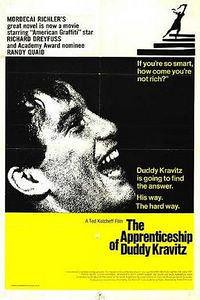The image is a vertical rectangular advertisement or movie poster taking up the entirety of the photo. It's designed to resemble the front cover of a book. The background features a gradient with sections of white, black, and yellow. 

At the top, against a white background, there are six lines of black text on the left side, which are difficult to read. There is an emblem on the right side, followed by four horizontal black lines that get progressively thicker towards the bottom. 

The central part of the poster has a black background featuring a man's head, possibly the star of the movie, Richard Drewes. The man, with short black hair, is looking up and to the right, seemingly smiling or laughing, though his face is cut off at the bottom. The black background also contains three lines of white print in the upper right and five lines in the lower right.

Towards the bottom, the background shifts to yellow. There is small black text in the center and, prominently on the right in blue print, the title "The Apprenticeship of Duddy Kravitz." The bottom right corner features three or four lines of very small black text, completing the detailed and layered design of this advertisement or movie poster.